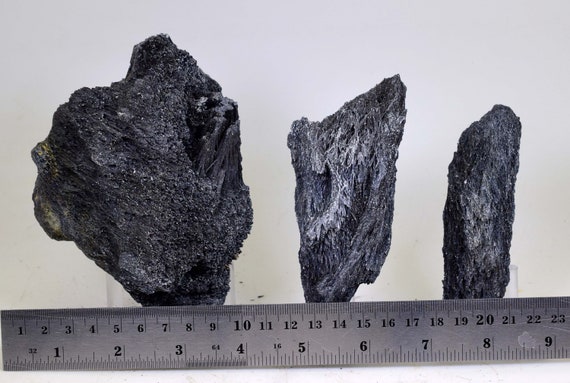This image depicts three dark gray to black volcanic rocks of varying sizes lined up against a metallic silver ruler on a white background. The largest rock, on the left, is the tallest and widest, characterized by its flat, porous, jagged surface, measuring roughly from the 0.5-inch to the 4-inch mark on the ruler. The middle-sized rock is about a third of the size of the largest, with a sharp, angular point and distinct light gray patterns, spanning from 5 inches to 6.5 inches. The smallest rock, resembling a rectangle in shape, is dark gray and extends from 7.5 inches to 8.5 inches. The ruler, a metal one that displays centimeters at the top and inches at the bottom, provides a clear reference for the size of each rock. The textures of the rocks are rough and highly detailed, with some shiny particles, potentially indicating metallic elements.